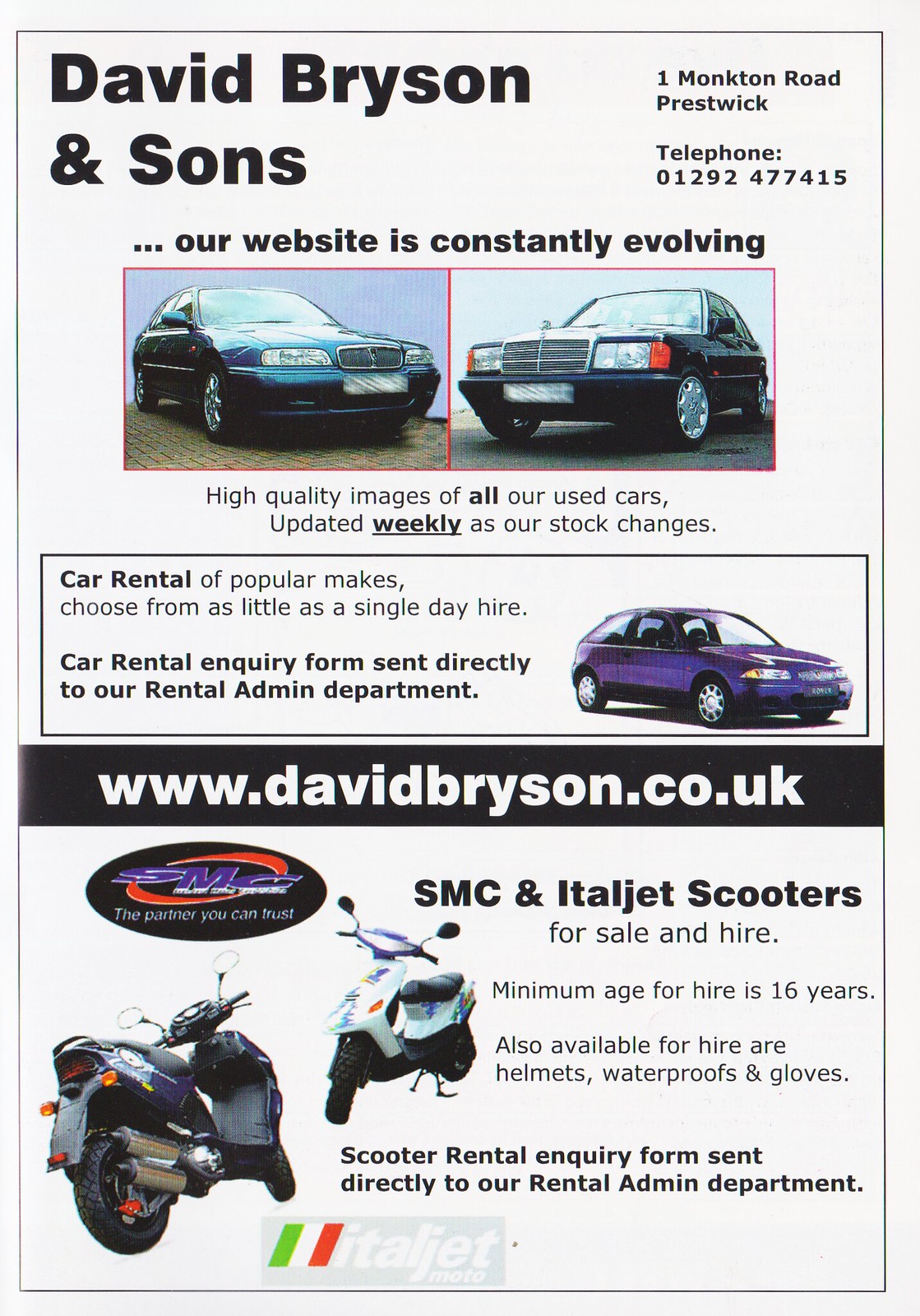This vertical advertisement features a clean white background with black text. At the top, in bold letters, it reads "David Bryson and Sons" followed by the address, "One Moncton Road, Prestwick," and a telephone number. The ad emphasizes that "Our website is constantly evolving" and provides the URL "www.davidbryson.co.uk" about halfway down the page. 

Below the header are two side-by-side thumbnail pictures of older cars—one teal and one black—forming a V shape. The teal car appears to be at the five o'clock position while the black car is at the seven o'clock position. A caption underneath these images states, "High quality images of all our used cars, updated weekly as our stock changes."

Further down, there is another image of a blue or purple car, facing roughly the five o'clock position, accompanied by more details about car rentals. Text in a bordered box highlights services related to "Car rental of popular makes," mentioning that rentals are available for as little as a single day and that an inquiry form is sent directly to their rental admin department.

Towards the bottom of the advertisement, on a black banner, the website URL "www.davidbryson.co.uk" is prominently displayed. Beneath this, there are pictures of two Vespa scooters with the label "SMC and Italian scooters for sale and hire." It provides information about additional items available for hire, such as helmets, waterproofs, and gloves, and specifies the minimum age for hire as 16 years. An inquiry form for scooter rentals is also mentioned to be sent directly to their rental admin department.